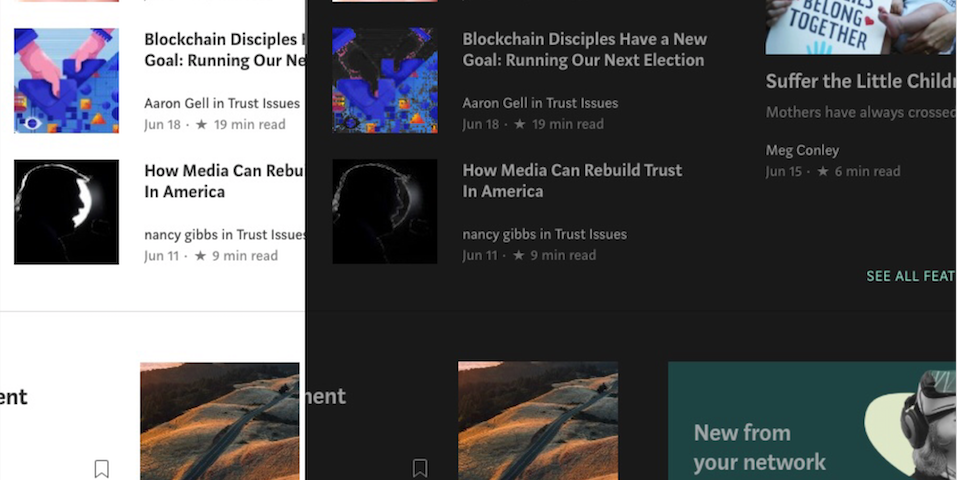The image is a composite of two overlapping screenshots featuring web search results. On the left side, there is a white section displaying two articles. The title of the first article is partially visible as "Blockchain Disciples..." but the rest is obscured by a large advertisement block overlaying it. The second article at the bottom includes a small landscape image depicting rolling hills with a road running through them. 

On the right side of the image, there is a prominent, black rectangular section containing several ads. One of these ads repeats the partially visible headline from the left: "Blockchain Disciples have a new goal, running our next election." This right section appears to be a superimposed layer, replicating elements from the left. At the right bottom corner, there is a label "New from your network" next to the same landscape image seen on the left.

Overall, the image is a blend of two screenshots with duplicated content, featuring articles, ads, and a scenic picture, providing a chaotic yet detailed visual of online search results and advertising overlap.